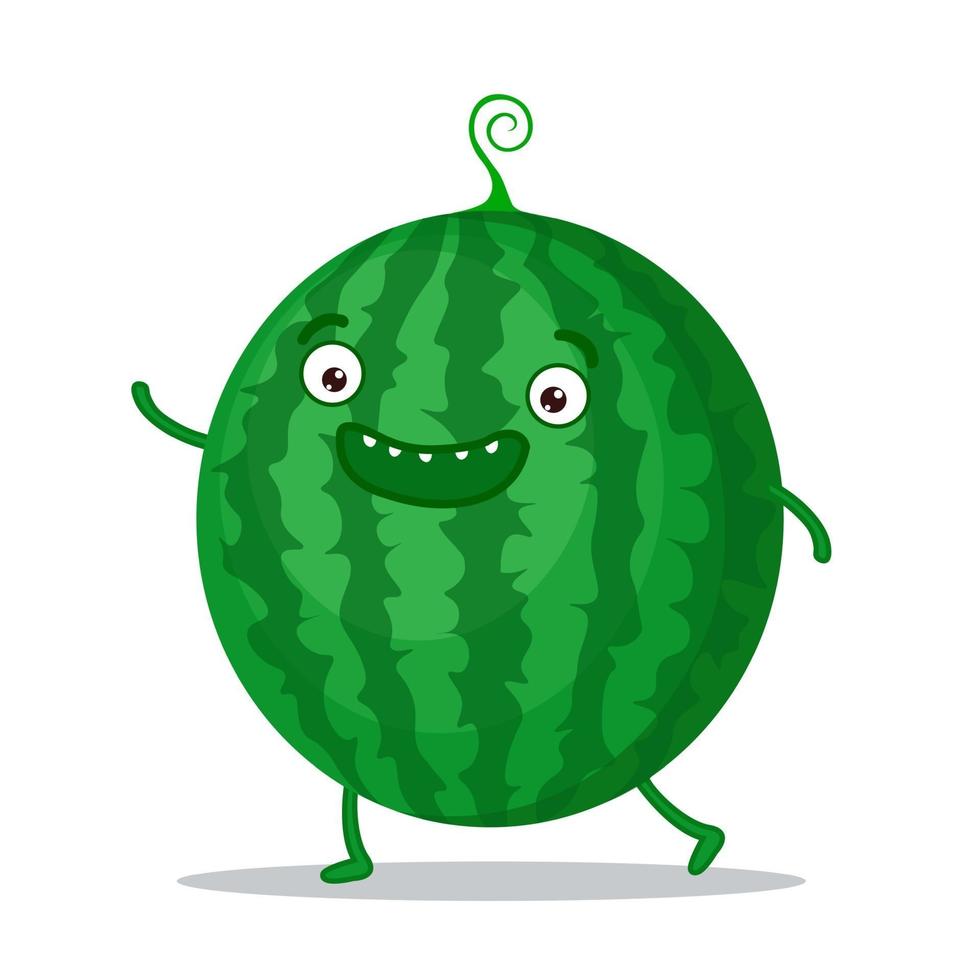In the image, there's a detailed and whimsical illustration of an anthropomorphized watermelon. The watermelon is distinctly round with a lively green hue adorned with dark green jagged stripes running vertically across its body. At the very top, a curly, tendril-like stem emerges, adding a playful touch. The watermelon features expressive white eyes with black pupils and dark green eyebrows set near the top of its body, enhancing its cheerful demeanor. Below the eyes is a wide, dark green mouth shaped vaguely like a sideways pickle, accented with small, white teeth on the upper row.

The watermelon is equipped with small, green limbs: two short, stem-like arms positioned in line with the mouth and two similarly styled legs at the bottom, which end in horizontal feet. It appears to be joyfully dancing, with its arms raised in the air. A soft, gray circular shadow is cast beneath the watermelon, grounding it against the plain white background. Overall, this digitally created piece captures the essence of a happy, animated fruit character bursting with personality.